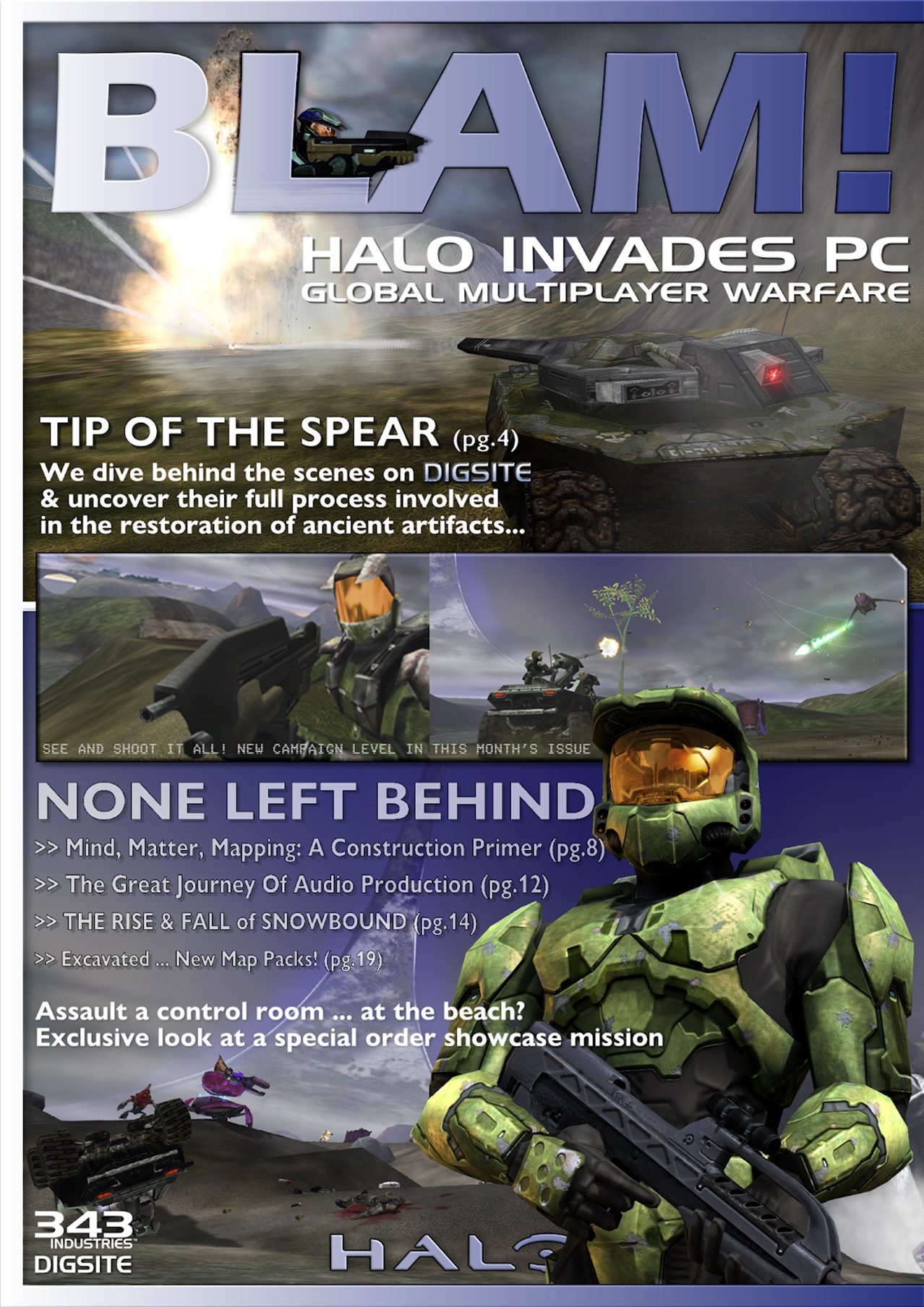BLAM! This visually striking magazine cover prominently features the title in gradient light to dark blue, standing out against a dynamic background composed of various images from the game. The cover highlights "Halo Invades PC Global Multiplayer Warfare" in bold white letters. Just above the title, amid the images, Master Chief, Halo's iconic character, is seen donning his signature green armor with a gold visor, holding an assault rifle.

A fireball explosion sets the energetic tone of the background, merging seamlessly with darker shades and a grey tank. The top section includes the headline "Tip of the Spear, page 4," inviting readers to explore an in-depth behind-the-scenes look at the Dig Site and its artifact restoration process.

The middle part of the cover features "None Left Behind, page 8," against a blue background. Below this, details about Mine Matter Mapping and a construction primer are provided, along with additional articles: "The Great Journey of Audio Production, page 12," "The Rise and Fall of Snowbound, page 14," and "Excavated: New Map Packs, page 19."

At the bottom, a digitally drawn soldier, resembling Master Chief in green armor and helmet, wields a black weapon. This section also teases an "Assault a Control Room at the Beach" scenario and offers an exclusive look at the "Special Order Showcase Mission." The cohesive blend of text and images creates a compelling visual narrative that draws readers into the multifaceted world of Halo on PC.